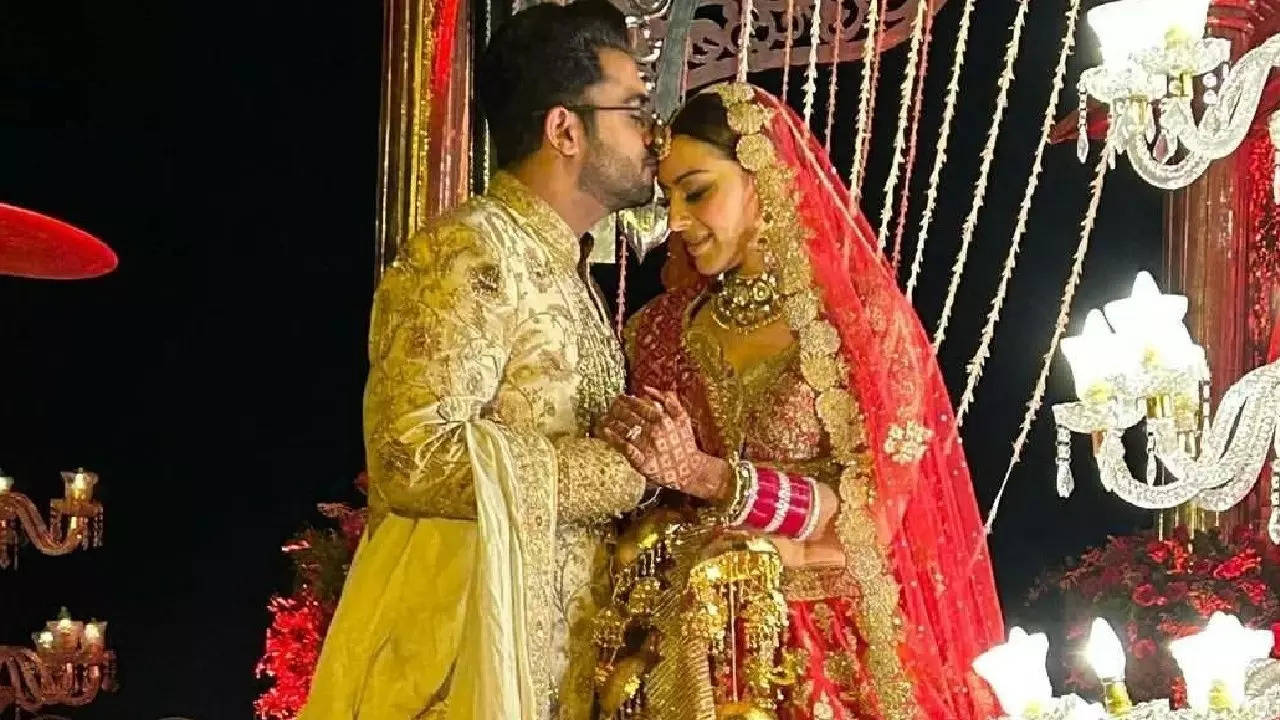This image captures an intimate moment at an Indian wedding, set against a pitch-black background, giving it a dramatic, almost stage-like quality. The young Indian couple, likely in their late 20s or early 30s, stand in the center, holding hands closely. The groom, positioned to the left of the frame, faces slightly right, at about 3 o'clock, while the bride, to the right, faces slightly left, at around 9 o'clock. The groom is dressed in an elaborate, gold-patterned traditional suit adorned with brown floral designs. He is also wearing glasses and tenderly kisses the bride's forehead. The bride, glowing in a long red dress richly decorated with gold accents, wears an equally ornate red veil trimmed with golden flowers. Her ensemble is further embellished with various golden jewelry and numerous red bracelets, while henna tattoos decorate her arms and hands. The photograph is richly adorned with sparkling star-shaped lights and dangling crystals, flanking the couple, adding to the luxurious ambiance of what appears to be a very special day.